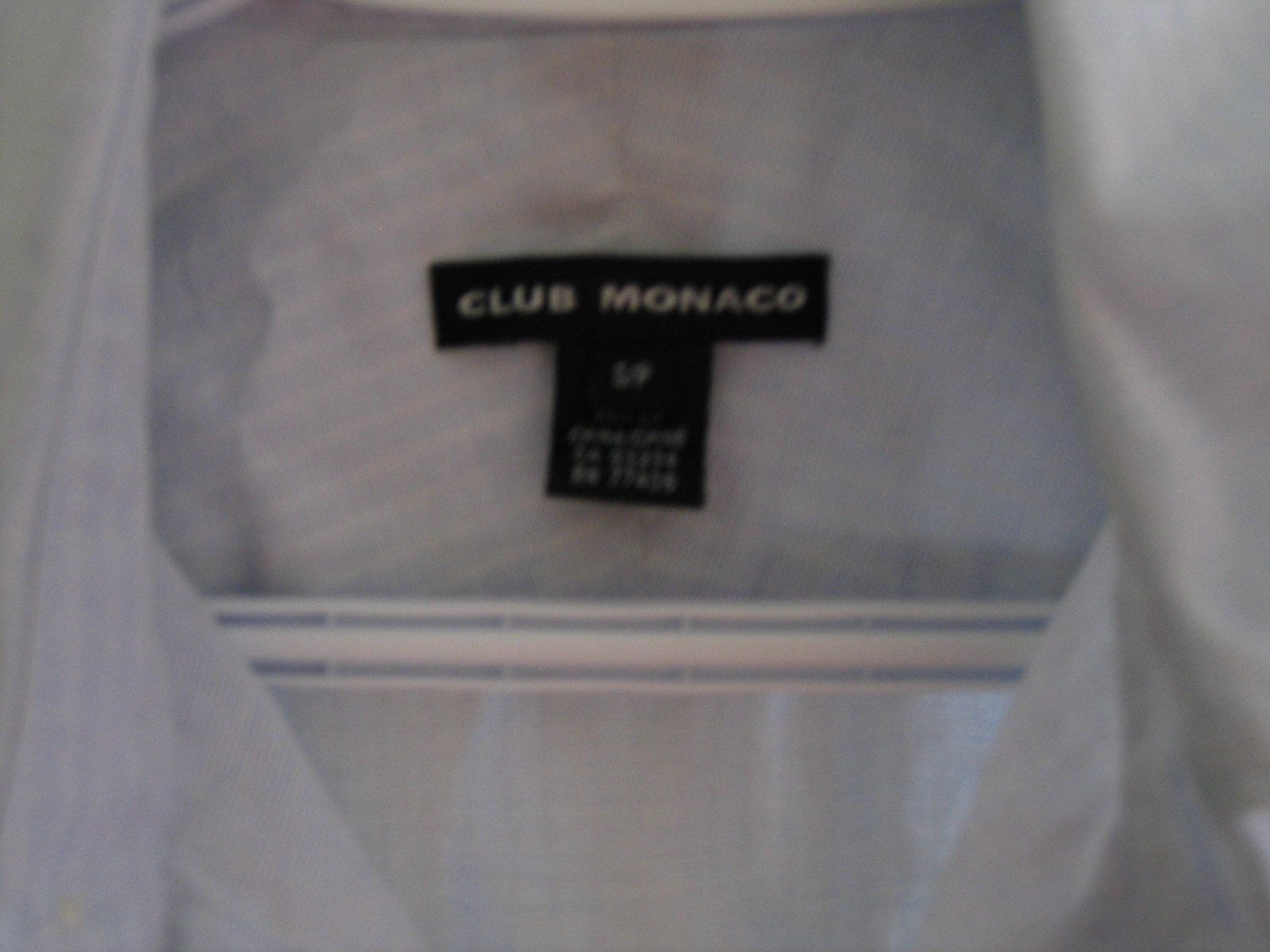A slightly blurred close-up photograph captures the inside tag at the back of a white button-down, collared shirt. The shirt features faint white stripes running through its fabric. It is hanging on a white hanger with two black lines running across it. Above the hanger, a small rectangular black tag is visible, displaying the brand "Club Monaco" in white lettering. Attached to this tag is a small square black tag with additional white writing that is indistinct due to the image's blur.